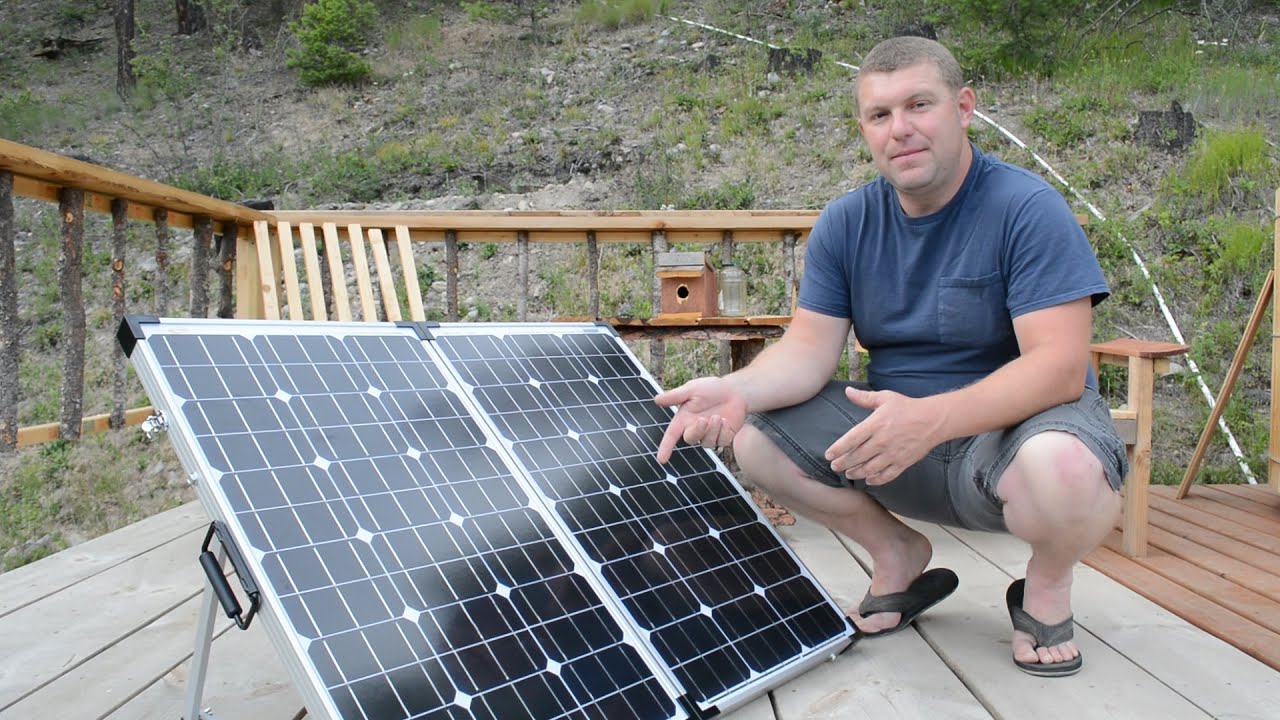In an outdoor setting characterized by a scenic greenery hill in the background, a man is seen crouching on a wooden deck. The deck, which appears to be part of a cabin or campsite, features a bird feeder on a bench. This man, with pale skin and short brown hair styled in a buzz cut, is showcasing a set of portable solar panels. He is dressed in a blue t-shirt with a pocket, knee-length gray shorts, and gray flip-flops. The man, who appears to be around 40 years old and heavyset, is squatting down and pointing at the black and white solar panels, which are opened and displayed prominently on the deck. The solar panels feature a handle hanging down from one side, indicating their portability. Behind him, the deck is adorned with a few objects including what looks like a birdhouse and a water bottle. The backdrop transitions from the wooden deck to scrubby grassland, adding to the natural and serene atmosphere of the scene. The man’s semi-smiling expression suggests a sense of accomplishment or excitement about the solar panels, possibly hinting at their use for generating power in this remote, wooded area.